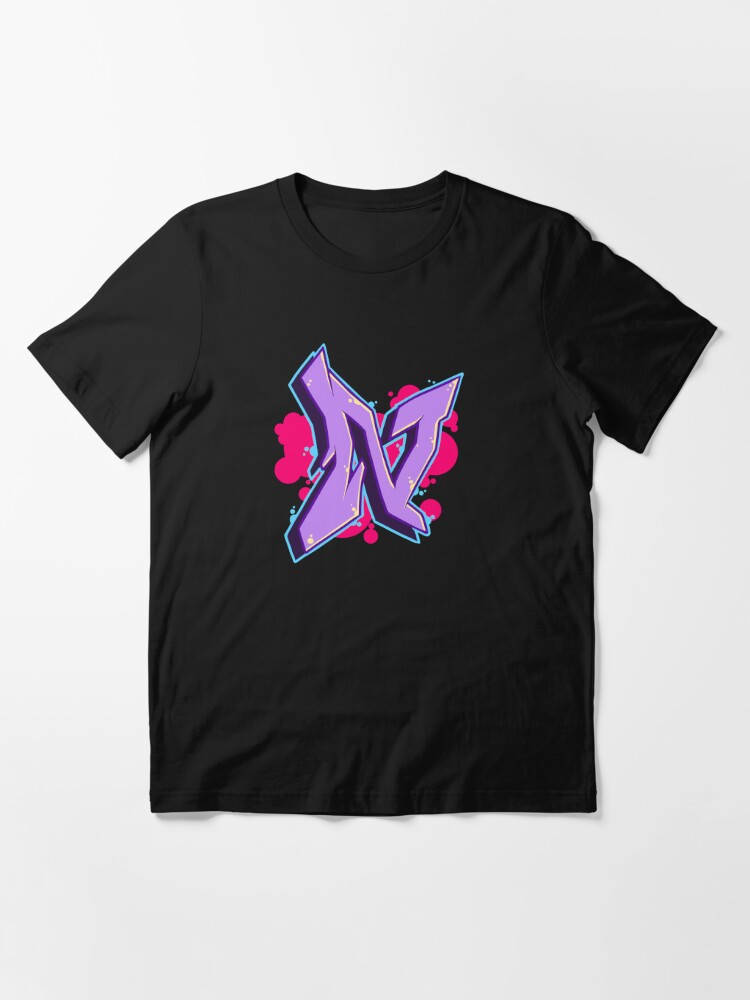This is a detailed photograph of a black short-sleeved, scoop-neck t-shirt with noticeable wrinkles, set against a grey background. At the center of the t-shirt is a prominent 3D graphic that most clearly resembles the letter "N" but could be interpreted as other characters such as "J," "V," "I," or even the number "7" due to its stylized, graffiti-like design. The graphic is primarily purple with a pink outline, accented by purple bubbles and light green bordering. The overall composition conveys a modern, somewhat abstract aesthetic.